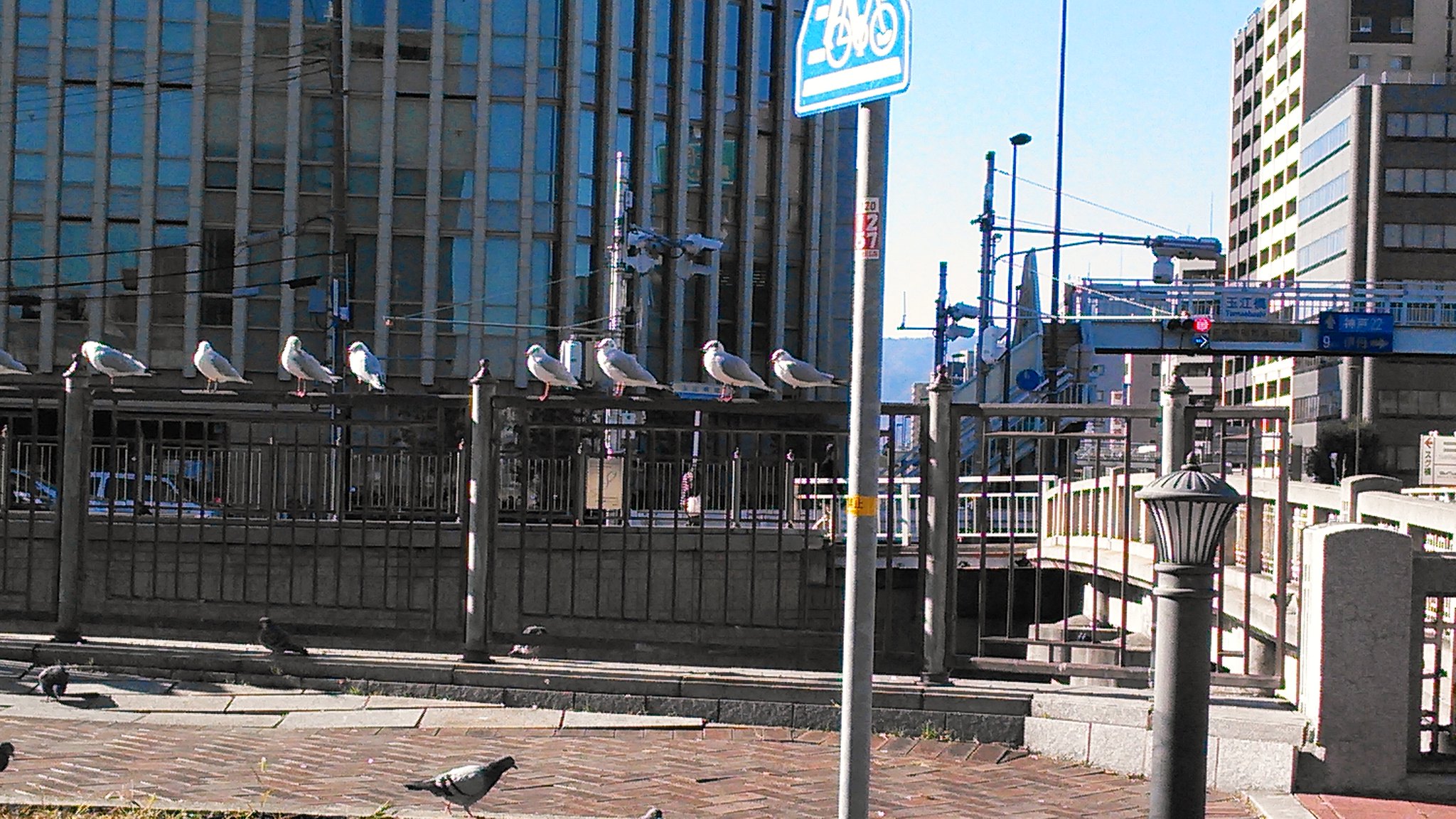In a bustling city, a group of eight pigeons perches on top of a metal barrier designed to prevent falls from a bridge. The railings consist of tall, silver rods bolted into the concrete and topped with round ends. Below, a few pigeons wander on a red brick sidewalk. A nearby metal pole adorned with stickers and a blue bicycle sign anchors the foreground. Behind this scene, a blend of large buildings, including a wide skyscraper filled with windows on the left and additional white and brown structures on the right, dominates the background. A metal pedestrian bridge spans a road, marking a lively yet tranquil urban setting. The photo captures the essence of a bright daytime moment in the heart of the city.